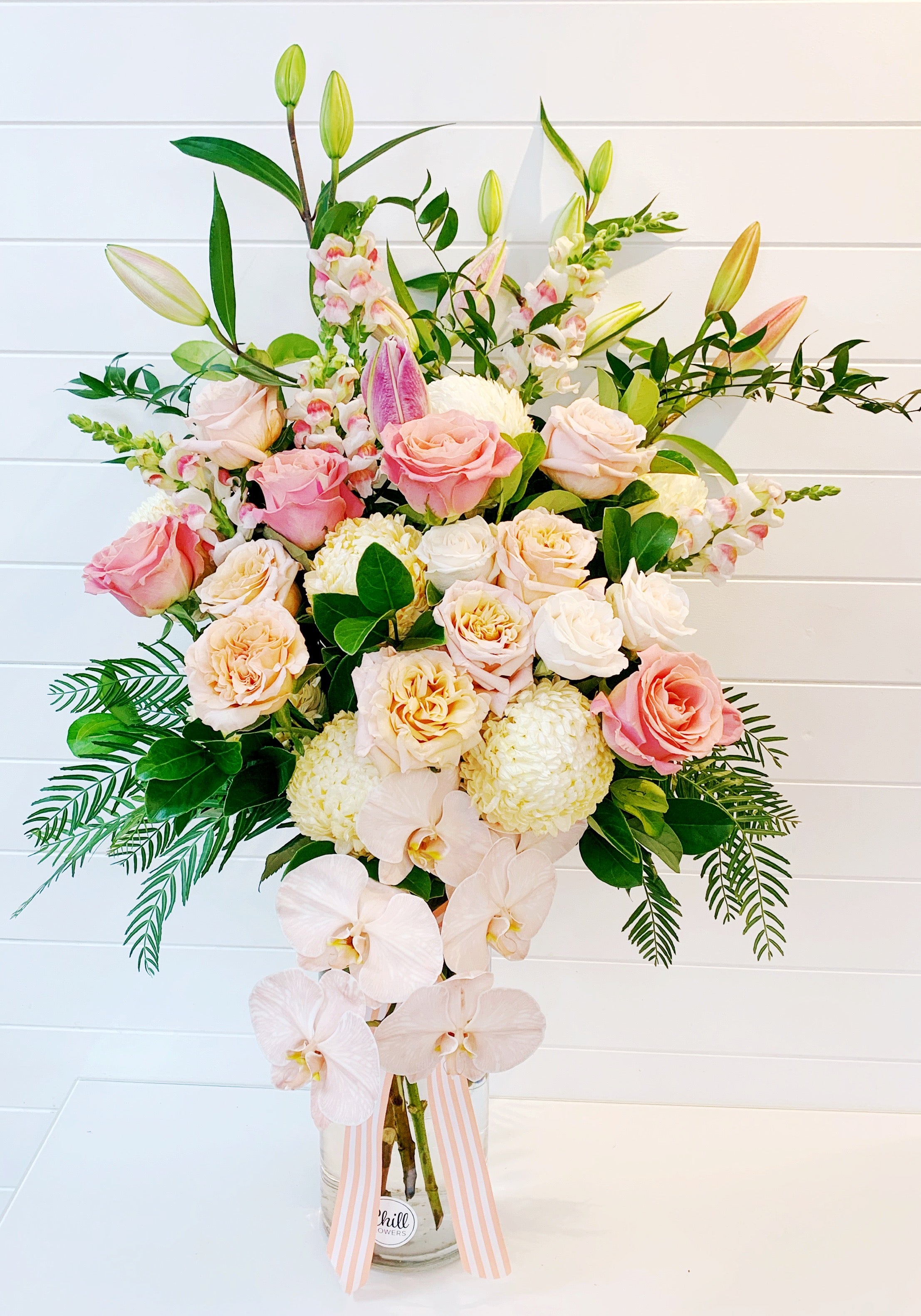This detailed photograph captures an intricately arranged bouquet designed for a celebration, possibly even a wedding. The bouquet is placed in a clear glass vase set on a white table, with a serene white background. The arrangement features a spectrum of roses: pale pink, medium pink, and deep pink, as well as a few peach-colored roses. Some roses are wide open, showcasing their yellow centers, while others remain as unopened buds. Adding to the bouquet's charm are big, fluffy blooms reminiscent of snowballs, likely hydrangeas, and smaller oval-shaped pink flowers. A few baby pink snapdragons rise elegantly towards the top.

The greenery consists of fern-like leaves and other foliage, complementing the colorful blooms and adding depth to the arrangement. Additional tall green plants with buds contribute to the bouquet’s vertical element. A striped ribbon in light pink and white is tied around the vase, enhancing the overall aesthetic. The stems of the flowers are clearly visible through the vase, grounding the vibrant array in its pure, transparent base.